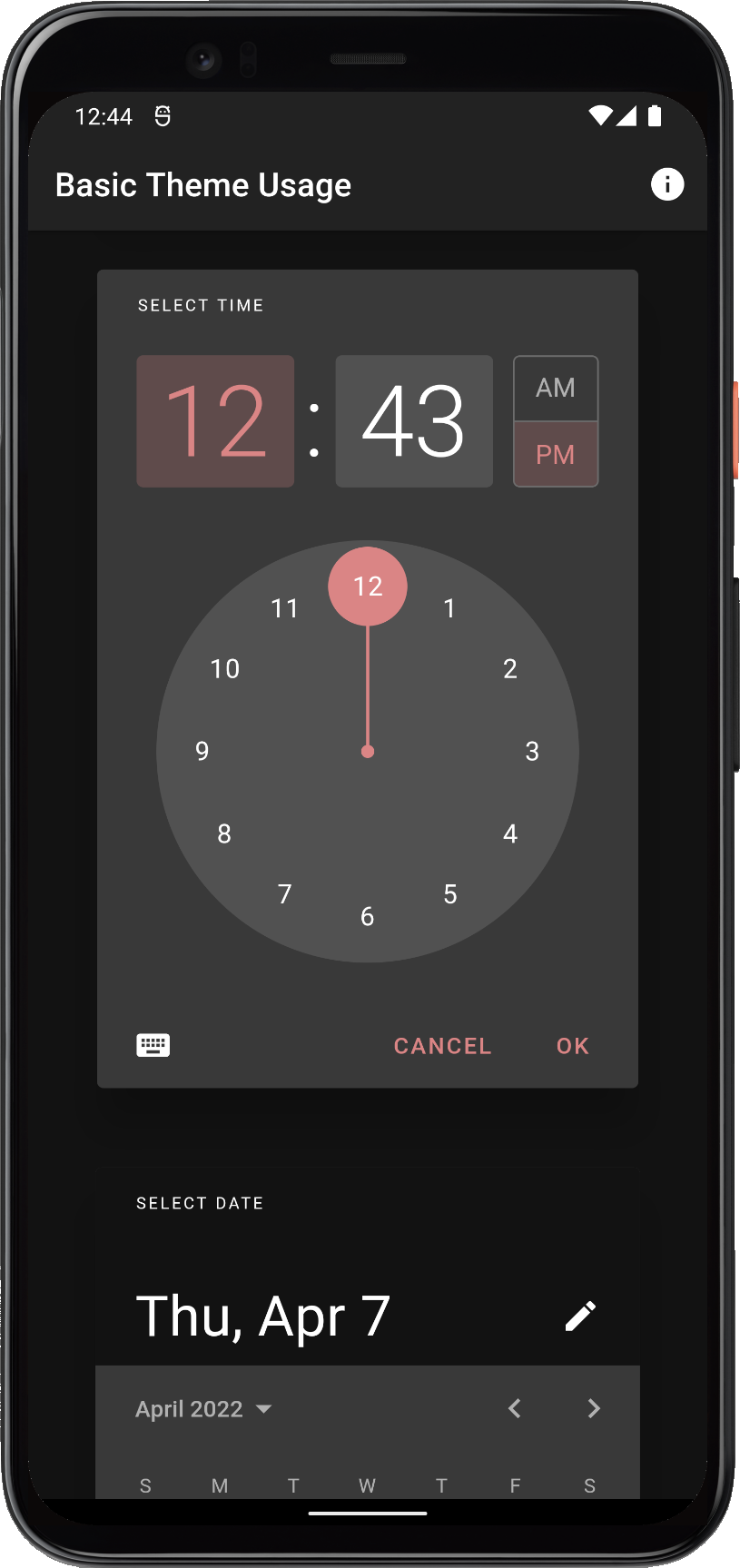A detailed screenshot of an iPhone app is displayed, which appears to be a time or calendar-related application. At the top of the screen, the header reads "Basic Theme Usage." Beneath this header, there is a functional interface labeled "Select Time," offering both digital and analog clock options for selecting a specific time. The screenshot shows that the time selected is 12:43 PM. 

Following the time selection section, there are two buttons: a "Cancel" button and an "OK" button, allowing the user to either confirm or cancel their chosen time. Below this section, a "Select Date" feature is visible, presented in calendar format. The date that has been tentatively selected is highlighted as Thursday, April 7th. Next to this date, a pencil icon is present, presumably for editing the selected date.

It is important to note that the full calendar view is not completely visible within the screenshot; the user would need to scroll down to access the remaining days of the month. Overall, the screenshot captures essential elements for setting a time and date within the app, but additional details are not displayed due to the limited screen view.